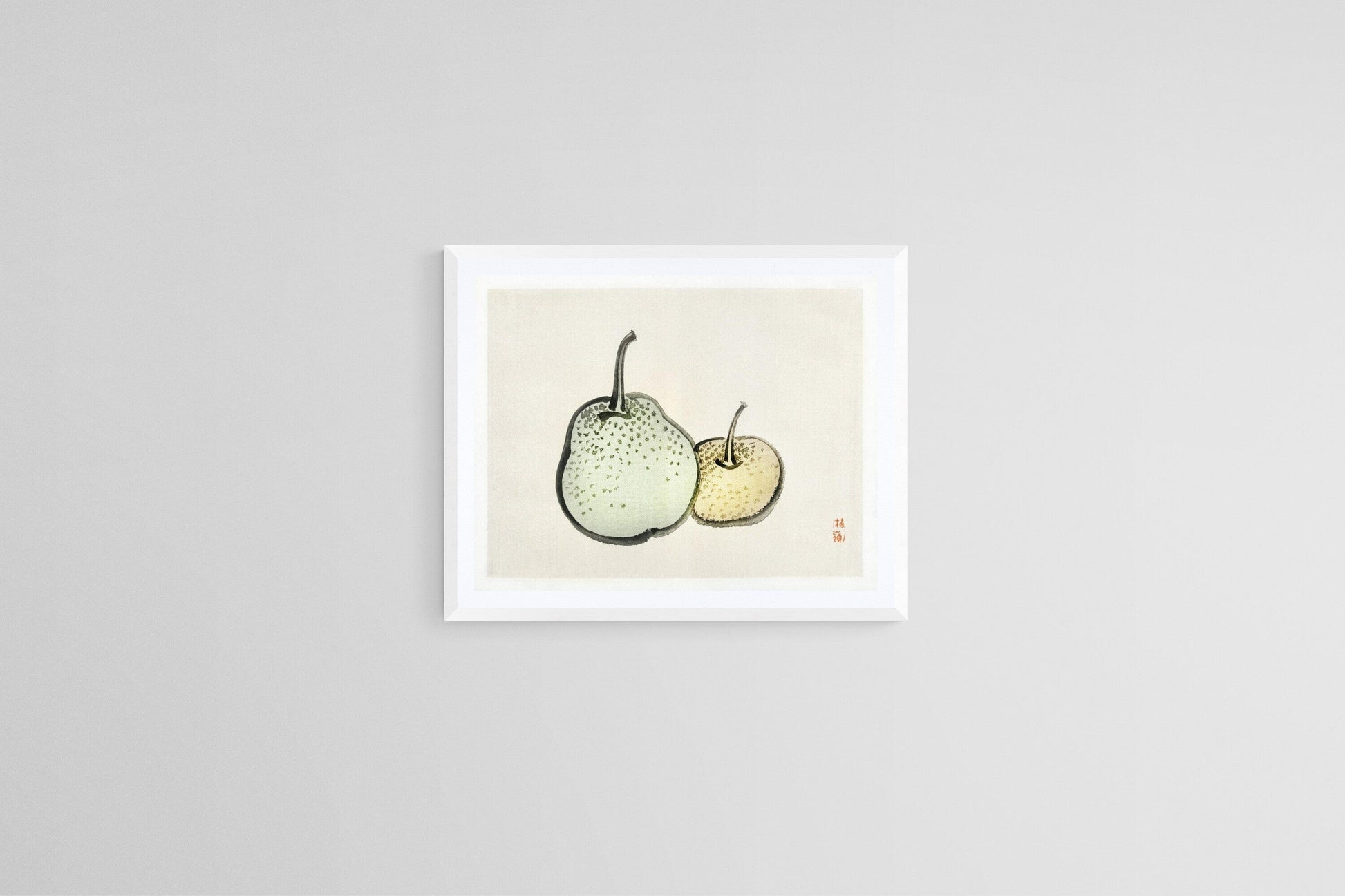The image depicts a simple watercolor artwork framed in white and displayed on a light gray wall. The white frame casts a faint drop shadow to the left and bottom. The artwork itself features a beige canvas with a pear and an apple-like fruit positioned centrally. The pear on the left is a very light, almost sage green color, adorned with tiny dark speckles that concentrate towards the top, accompanied by a thin black stem. The fruit on the right resembles an apple or peach with a light yellow hue, marked with light brown spots, and also has a thin black stem. Both fruits are outlined in a thick, watercolor black that gradually fades to become more transparent on the right side. In the bottom right corner of the canvas, there's a small, red signature from the artist, although it's too small to be legible from a distance.